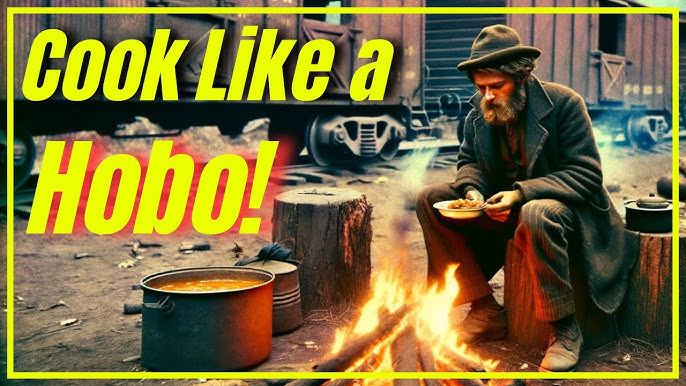The poster features a rectangular photograph, bordered by a thin yellow line, and adorned with bold, two-line yellow text in the upper left corner that reads "Cook Like a Hobo!" with "Hobo" emphasized in larger letters with red shadowing and an exclamation mark. The scene depicts a hobo sitting on a tree stump in front of a small, orange-yellow campfire, holding a white ceramic bowl filled with stew. He is dressed in a gray overcoat, a dark shirt, dark brown striped dress slacks, worn shoes, and a dark hat with a small brim. His gray beard and mustache frame his weathered face. To his left is a large gray metal pot, brimming with yellowish soup and situated near a coffee can and another pot on a separate tree stump. In the background, a line of reddish-brown railway cars stretches across the image, with one featuring an open door. The ground is a mix of dirt and scattered leaves, emphasizing the rustic setting.